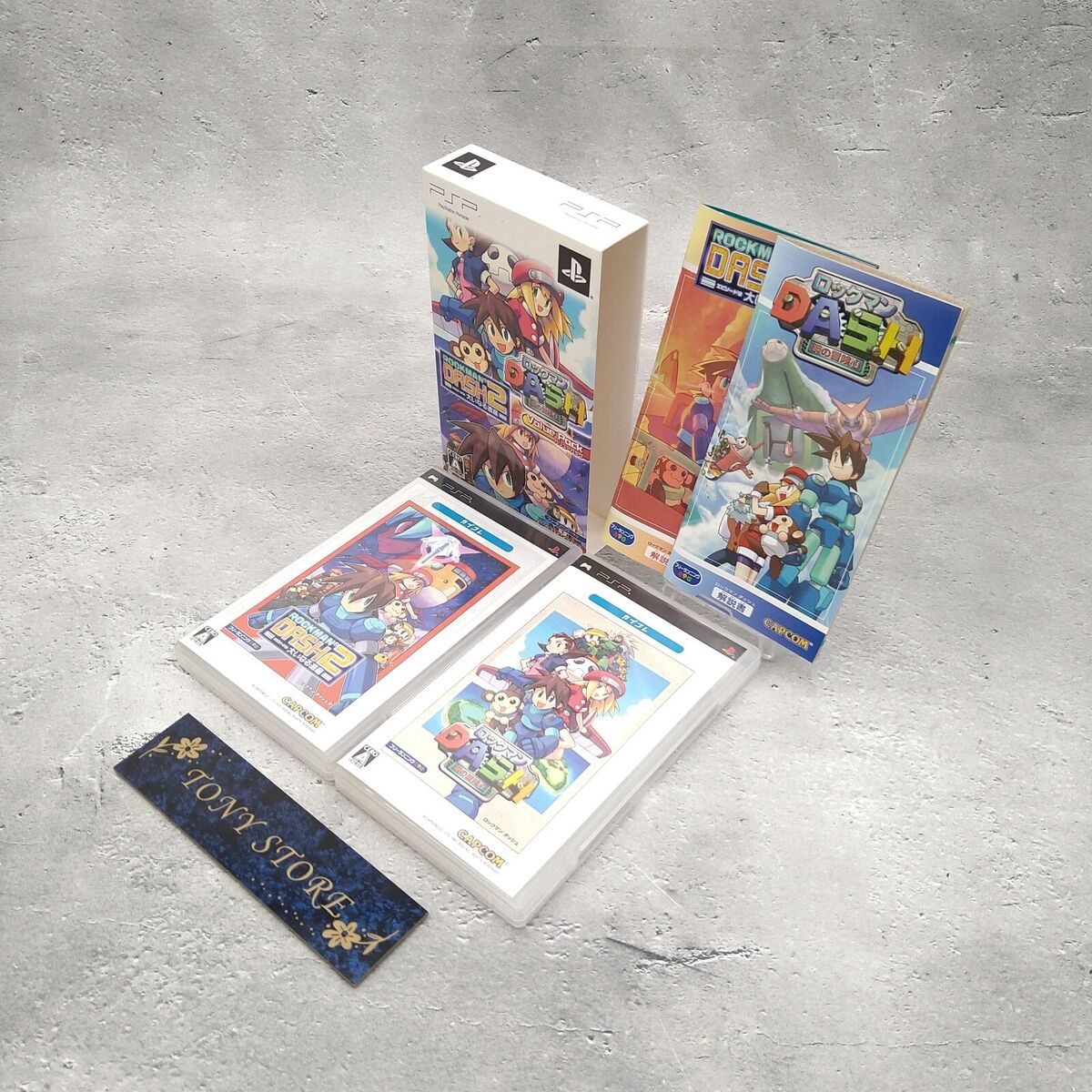In this promotional photograph for a Japanese video game by Capcom titled "Dash and Rockmaster Dash," the scene is meticulously arranged to display the game's complete contents. The image showcases several game cases for the PSP, laid out on a rugged, gray concrete floor riddled with pits and scratches. The backdrop shares the same gritty concrete texture, enhancing the staged setting. Positioned at a slight angle, two video game cases lie at the forefront, while an additional game box sits above, slightly open to reveal colorful covers of multiple titles leaning against a plastic holder. The vibrant game covers feature characters with prominent, expressive eyes. A distinctive blue name tag adorned with brown flowers in the top left and bottom right corners, and displaying the gold text "Tony Store," is prominently placed below the video game cases, presumably indicating the store selling these games.